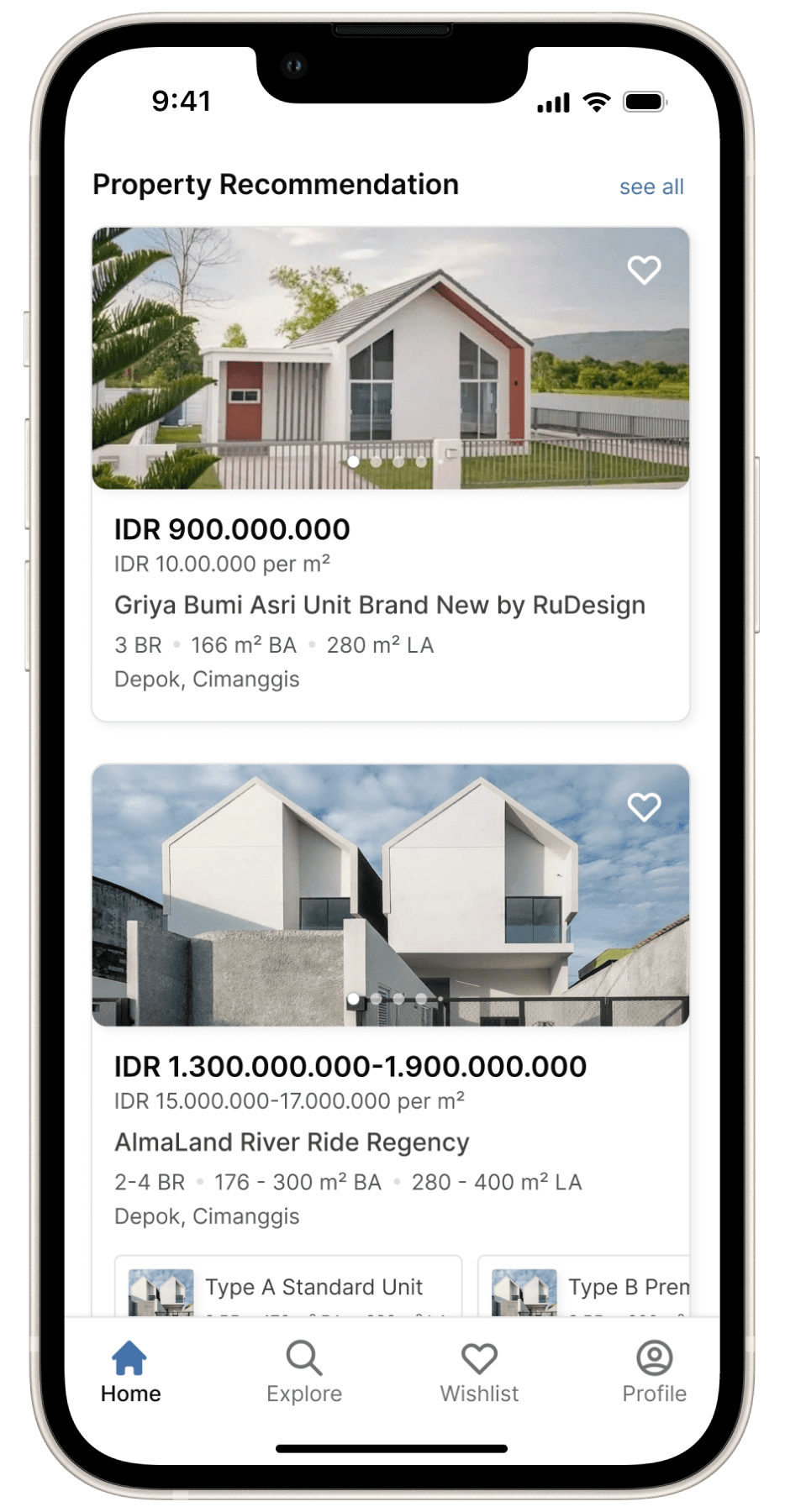This descriptive caption details an image featuring a screenshot from a smartphone:

The screenshot displays a cell phone screen framed by a black border. At the top left, the time is shown as 9:41, while the top right features three fully charged icons: signal strength, Wi-Fi strength, and battery strength, all depicted in black. Below these indicators, a real estate app is in use, showcasing property recommendations.

The main heading reads "Property Recommendation" in black text, accompanied by a "See All" link on the right. Below this heading, two property listings are displayed.

The first property listing includes an image of a small house surrounded by trees. To the right of this image is a heart icon for bookmarking the property. The details below the image state the price as 900 million Indonesian Rupiah (IDR), with a rate of 10 million IDR per square meter. The property is a unit in "Gria Bumi Asiri," designed by Rue Design, and includes specifications such as the number of bedrooms, square footage, and bathrooms. It is located in Depok, Cimanggis.

The second property listing features an image of modern, two-level condos. Similar to the first property, the price is listed in Indonesian Rupiah, with design and location specifics provided. This unit is part of the "Almalan River Ride Regency," with details on the number of bedrooms, square footage, and its location in Depok, Cimanggis.

At the bottom of the screen, four navigation buttons are visible: Home, Explore, Wishlist, and Profile.